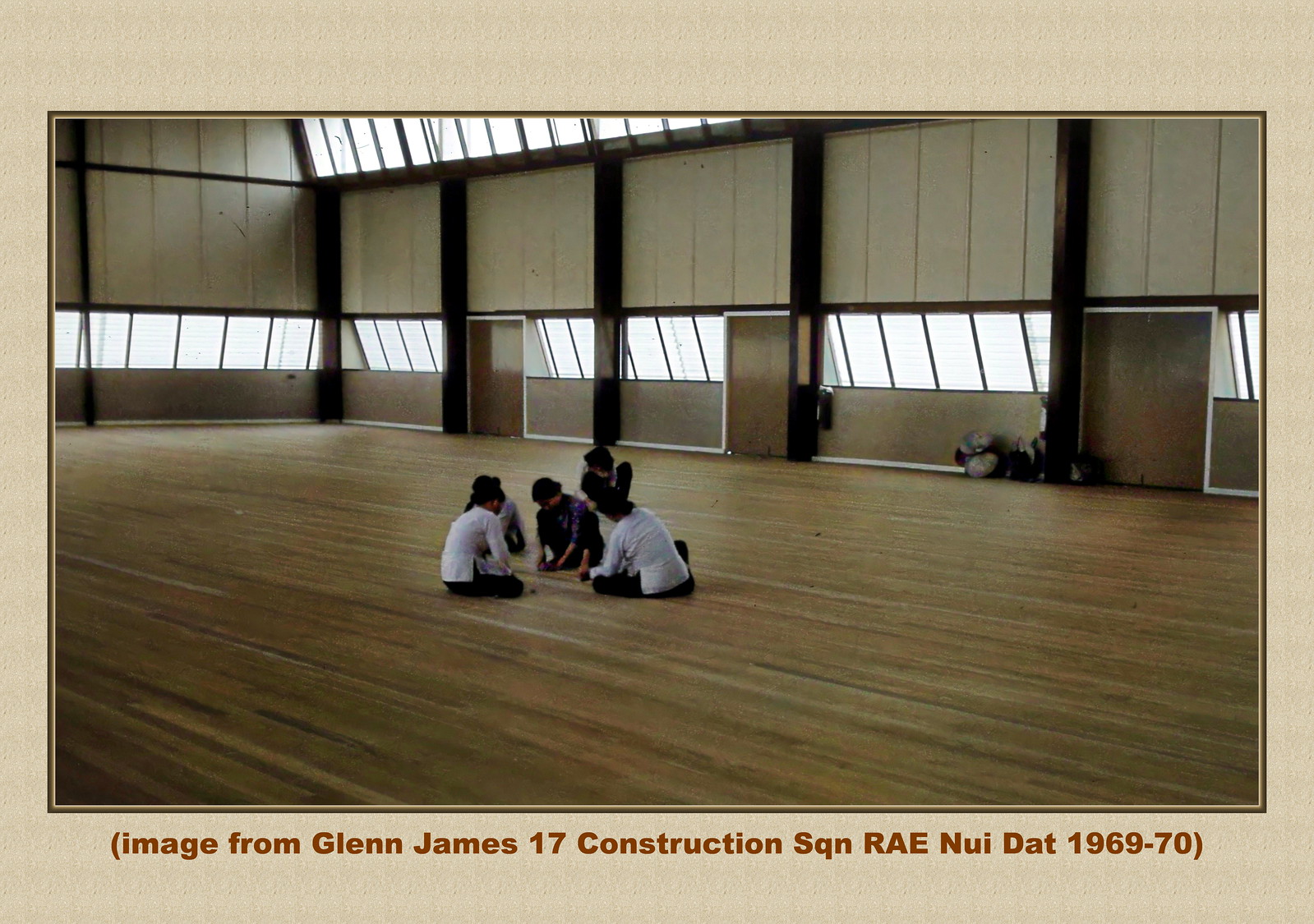This detailed image captures the interior of a gymnasium illuminated by light streaming through numerous windows, both in a lower row and higher up. The gymnasium, characterized by its brown wooden floor, brown doors, and a mix of light brown and white on the walls, also features black support beams. Central to the photograph, five individuals, possibly children, sit cross-legged on the floor, seemingly engaged in an activity though it’s not clear what. Two of them wear white t-shirts with black pants, while the others appear to be in black attire. Around the edges of the image, notably near one of the doors, several backpacks are visible against the wall. The photograph is bordered in a light tan color and beneath it, a caption reads, "Image from Glen James, 17 Construction Squadron, RAE, New Dat, 1969-70."